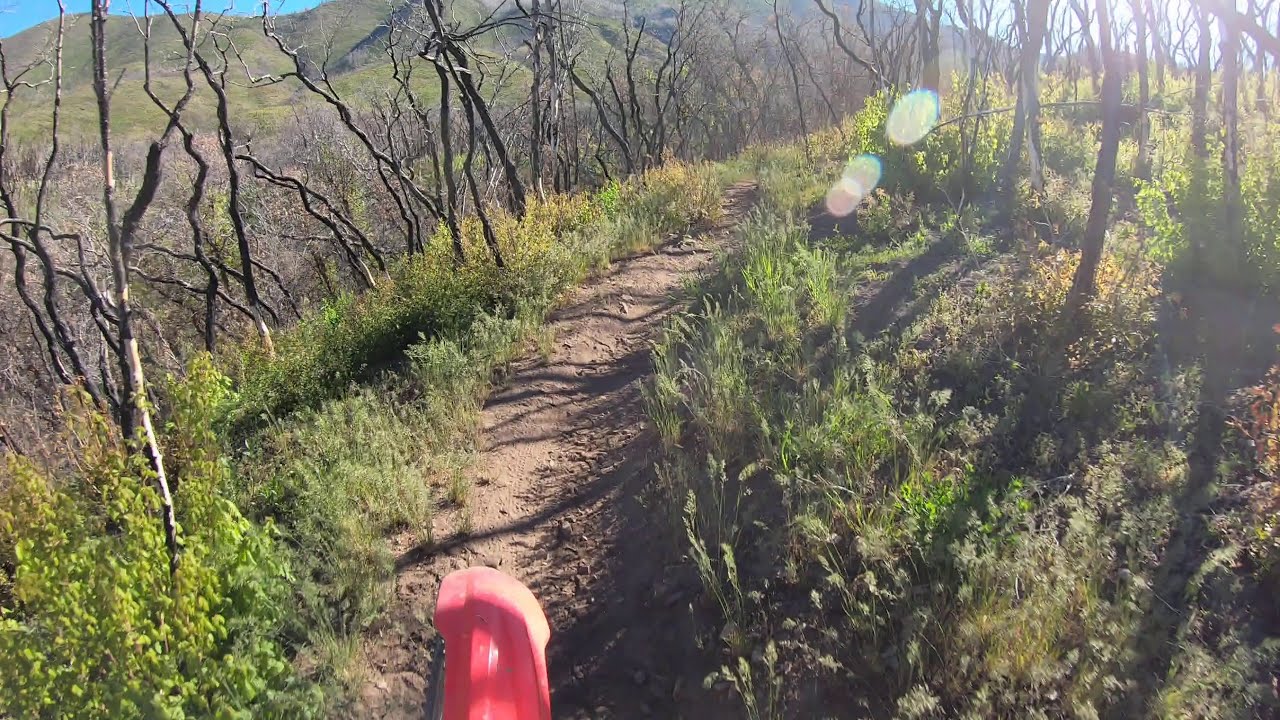A picturesque hiking trail winds its way through a rural, mountainous area under the bright mid-day or early evening sun, which casts long shadows on the surrounding terrain. The narrow dirt path curves gently to the right, cutting through an undergrowth of green grasses and low shrubs. Leafless, thin trees and tall, lifeless plants line both sides of the trail, their bare branches reaching skyward. In the distance, a range of majestic mountains provides a stunning backdrop, shrouded in shades of green and gray. At the bottom of the image, partially obscured, is a pinkish-red, slightly orange plastic object resembling the letter "B." Near the top left and middle left of the scene, two large, transparent grayish spots on the camera lens—likely water droplets—create a soft, oblong distortion, adding an ethereal quality to the image. There's also a hint of a motorcycle tire and motor guard visible, suggesting the trail is being explored by a rider, though no person is in view.